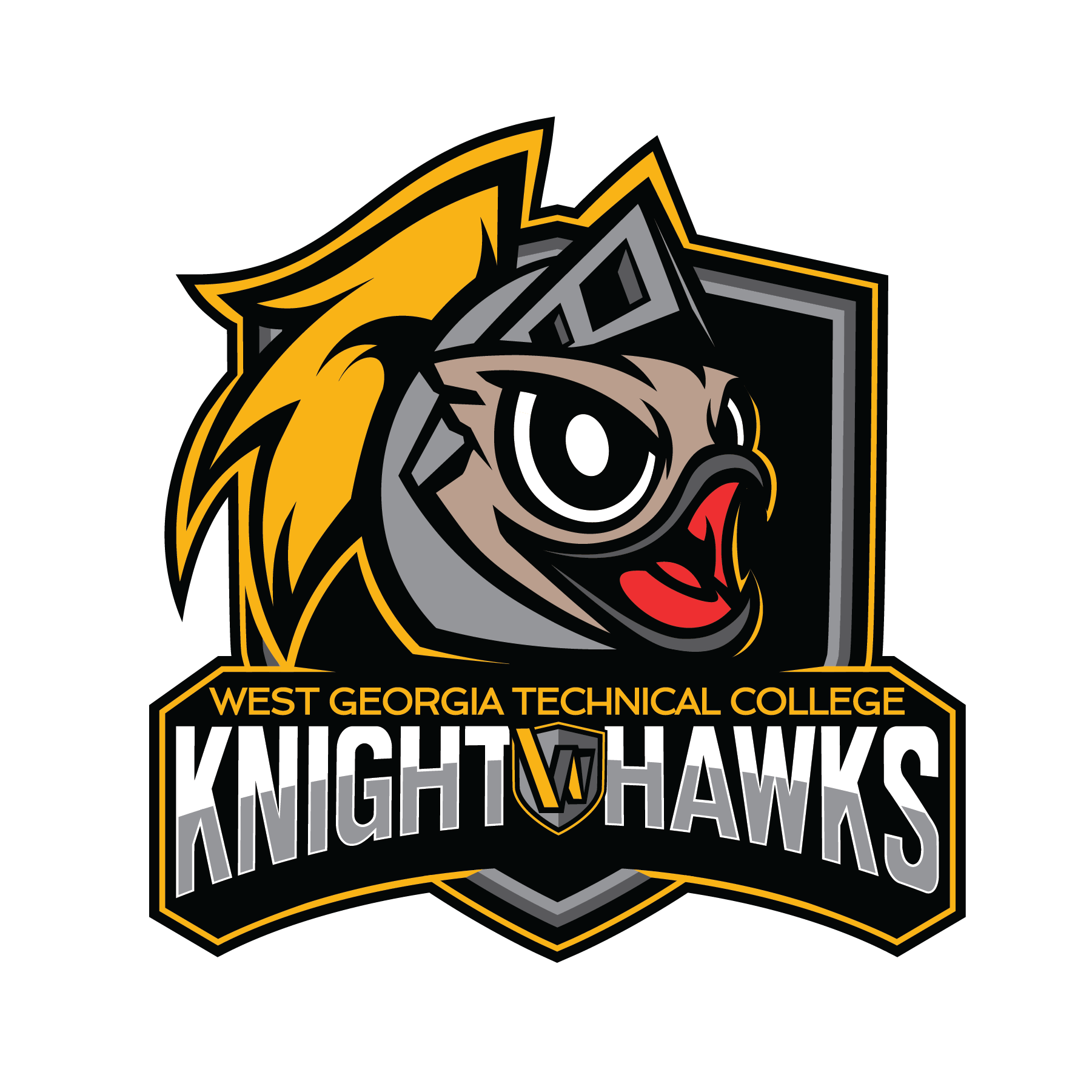This full-color, computer-illustrated flat vector logo represents the West Georgia Technical College Nighthawks sports team. The central figure is a cartoonish hawk mascot wearing a knight’s helmet, which is silver with an orange feather protruding from the top. The hawk has a light brown face, a wide-open black beak revealing a red interior, and large black-and-white eyes. Surrounding the mascot is a black shield with an orange border. An arched banner at the bottom of the image reads "West Georgia Technical College" in orange letters on a black background, and "Knight Hawks" in a stretched-out gray and white font. The logo combines elements of both knight and hawk imagery, encapsulating the team’s spirit and identity in a dynamic and engaging design.